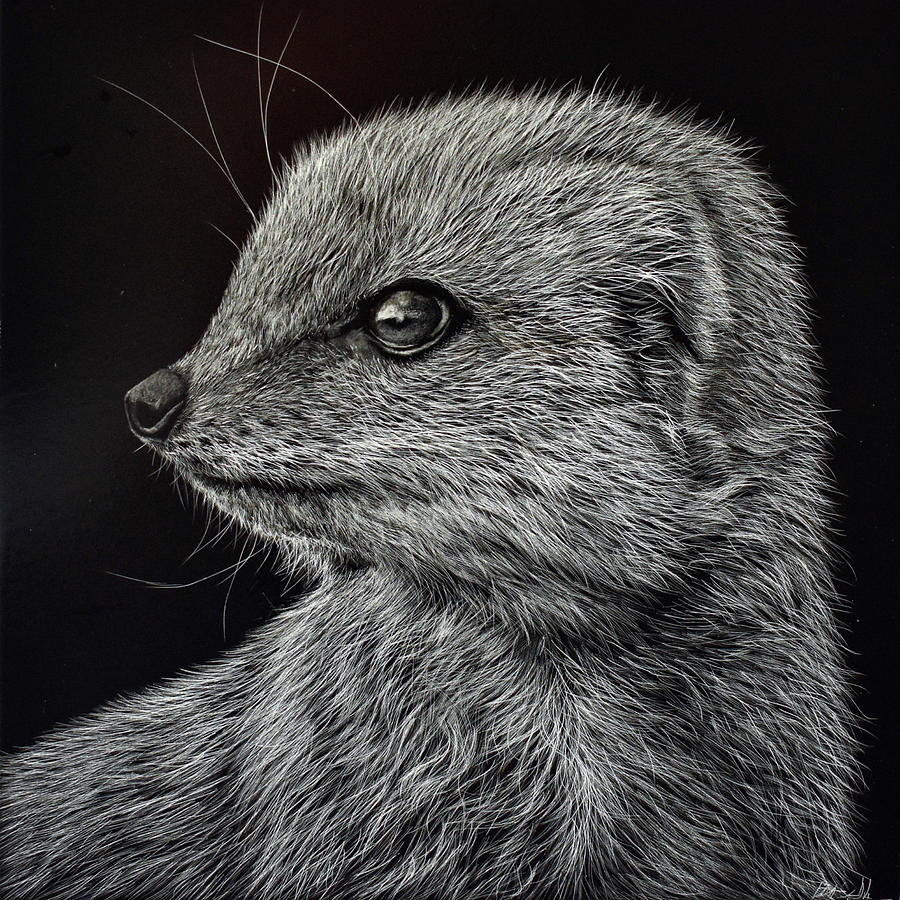The image presents a highly detailed, black-and-white representation of a rodent-like mammal, possibly resembling a hybrid of a mole, meerkat, or squirrel, though its exact species is indeterminate. Captured or rendered in a style so realistic that it appears photorealistic, the creature stands out sharply against an entirely black background. It is shown from a side profile, with its body visible from the chest up, seemingly standing on its hind legs and looking intently towards the left. The mammal's fur is predominantly white, interspersed with some black hairs that create subtle shadows, particularly around the eyes and snout. Its eyes are shiny and iridescent, with a slight light reflection, adding a lifelike quality to its gaze. Prominent, tall whiskers jut out from its snout and above its mouth, enhancing its detailed, furry appearance. The fine textures of the fur and the creature's poised stance contribute to the intricate and captivating visual. At the bottom right, a signature hints at the image’s artistic origins, confirming it as an illustration.